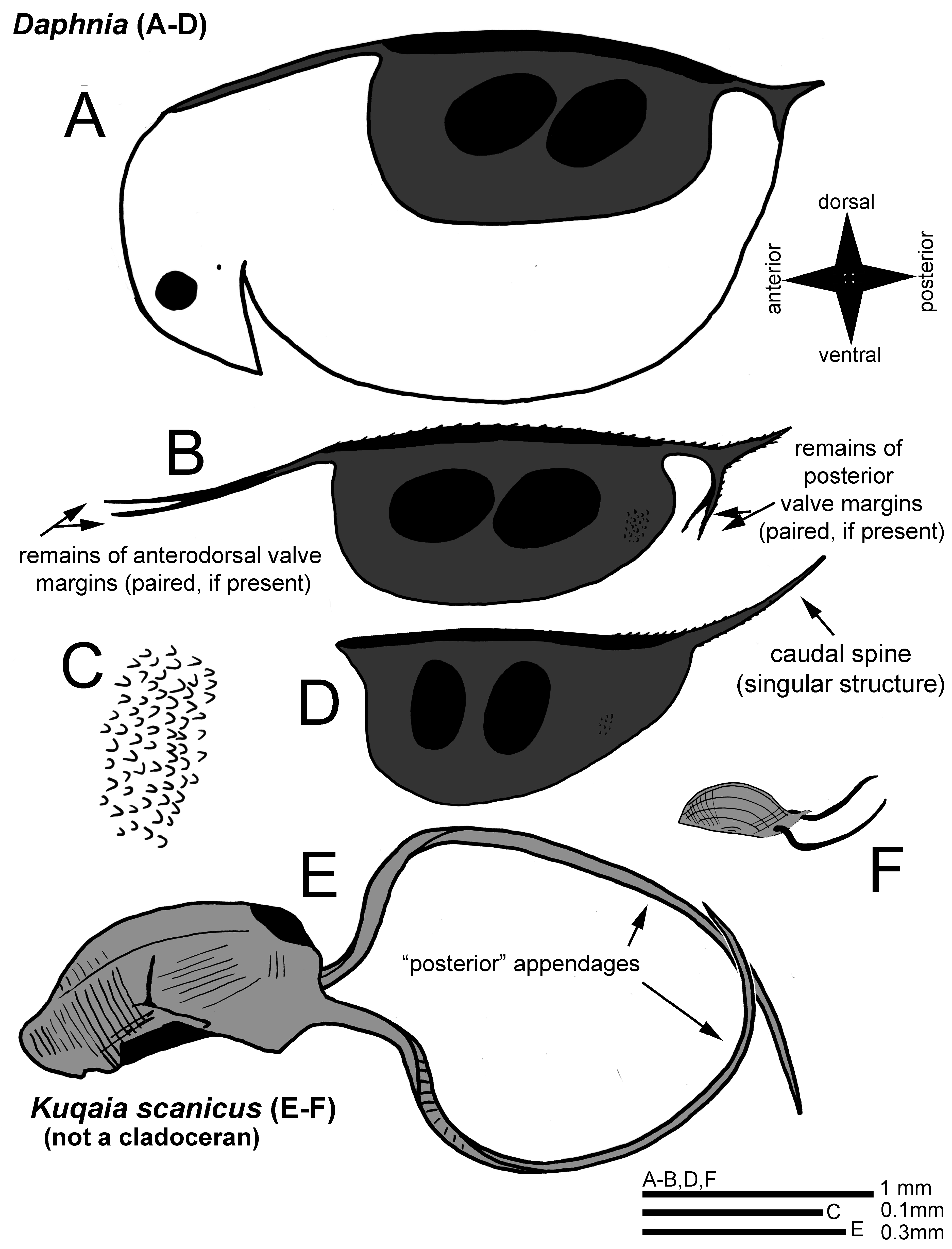The image appears to be an educational chart illustrating various parts of Daphnia, labeled A through F, and includes a star compass indicating orientation: dorsal (top), posterior (right), ventral (bottom), and anterior (left). Label A, resembling a sideways bird, features the main body with a star compass for orientation. B focuses on the darker anterior or dorsal valve margins, paired if present, and the posterior valve margins. Label C depicts numerous squiggles, possibly representing smaller structures or cellular fragments. D shows a caudal spine, labeled as a singular structure. E and F (collectively identified as quokkaeus scannuus) depict posterior appendages, with E looking like a vacuum cleaner with legs and F showing a simple outline. The chart includes measurements at the bottom, with labels A through B, D, and F indicating sizes ranging from 0.1 millimeters to 0.3 millimeters.